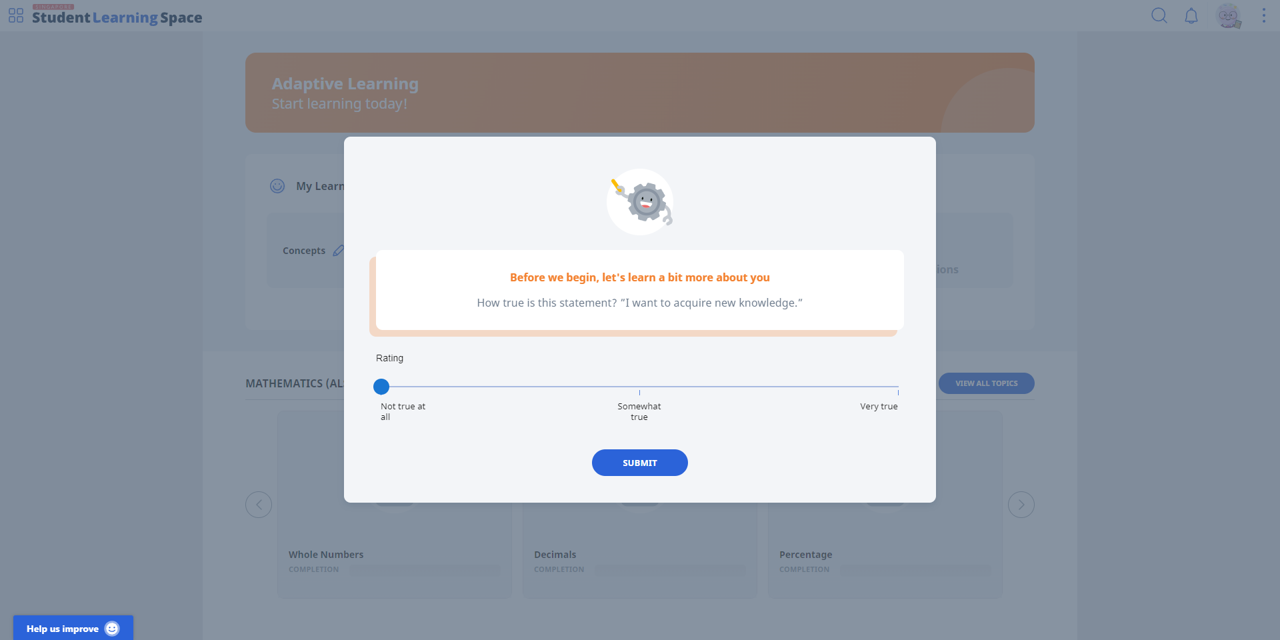In the image, there is a grayish pop-up box with rounded corners. At the top of the box, there is a small illustration featuring a friendly gray gear character with a smiling face, holding a yellow pencil. The gear character is placed within a white circle. Below this illustration, the box contains a heading in orange text that reads, "Before we begin, let's learn a bit more about you." 

Underneath the heading, a gray text box asks, "How true is this statement? I want to acquire new knowledge." A rating bar is provided with a movable blue dot that allows users to select their agreement with the statement. The options range from "Not true at all" on the left, "Somewhat true" in the middle, to "Very true" on the right. Currently, the blue dot is placed at "Not true at all." 

Beneath the rating bar, there is a blue "Submit" button. The background of the page is slightly grayed out, with the header displaying "Student Learning Space" in the top left corner. An orange box labeled "Adaptive Learning, Start Learning Today" is also visible. In the top right corner, there are icons for a magnifying glass, a bell, and a profile picture.

Additionally, there are several boxes with educational topics such as "Mathematics," "Whole Numbers," "Decimals," and "Percentage." In the bottom left corner, a blue box with the text "Help us improve" and a smiley face is displayed.